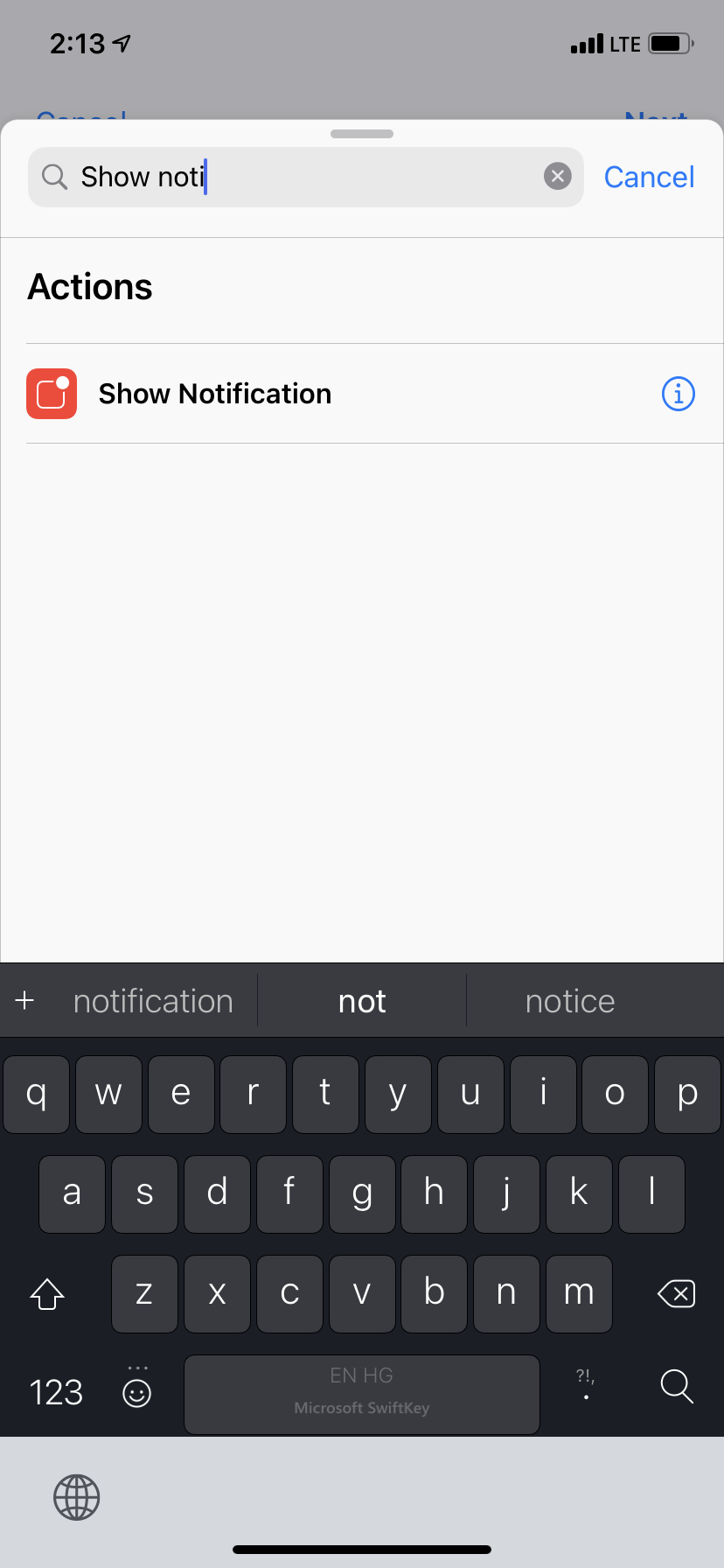A smartphone screen is displaying a webpage, indicated by the battery icon, signal strength bars, time code, and LTE symbol in the upper right-hand corner. The webpage features an interface where a user has activated a notification action. The search bar at the top contains text and is accompanied by a highlighted "Show Notifications" option, marked with a black font. Below this, the word "Actions" is displayed in a larger black font.

The lower portion of the screen shows a virtual keyboard, standard for texting, with black keys and white letters. This keyboard is offering word suggestions based on the user’s input in the search bar. Additionally, a cancel button is positioned next to the search bar, enabling the user to discard the notification process if desired. In the bottom left-hand corner of the screen, a globe icon is present, hinting at language or global settings options.